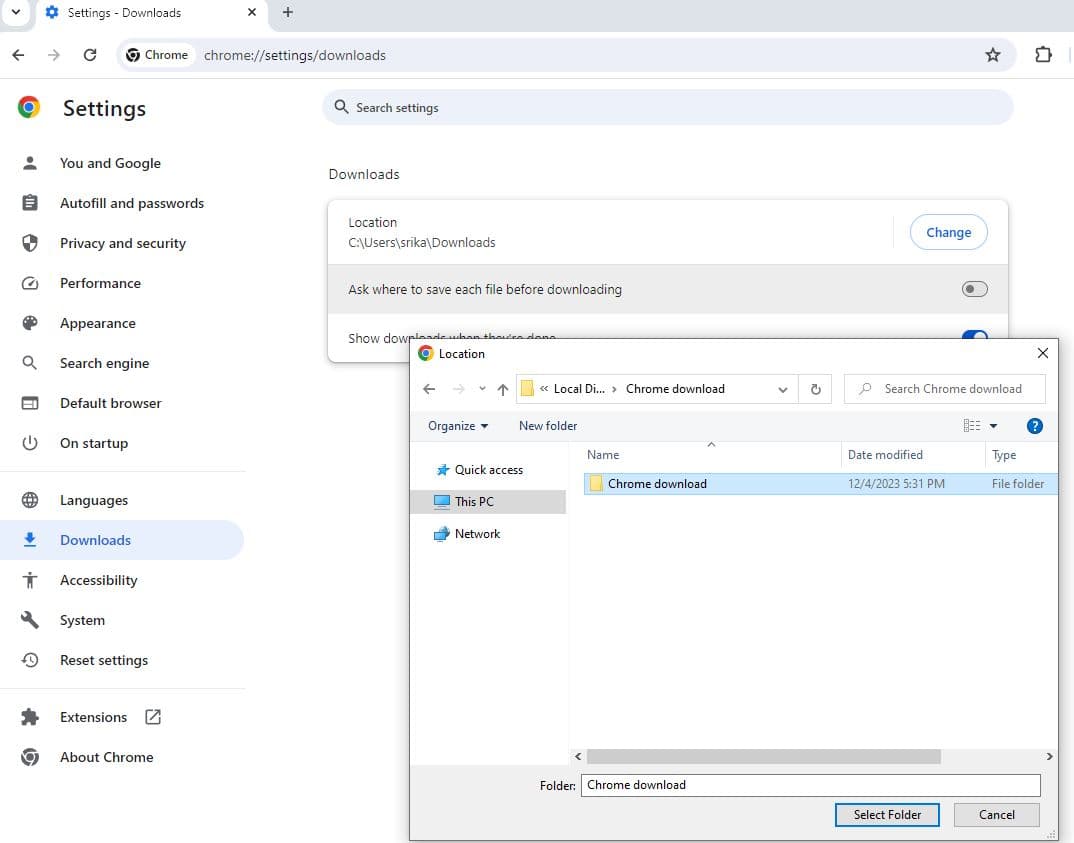A screenshot of a Chrome browser settings page is displayed. The user is in the "Downloads" section, with an option highlighted to change the download location. The current download folder is set to "C:\Users\Srika\Downloads", and they are about to change it to "Chrome Download" within the "This PC" directory on the D drive. The browser window shows only one tab open, which is the settings tab. The interface includes a search bar at the top. The overall color scheme of the browser is gray, with white used for the tab and page background. Two pop-up windows are visible: one showing the current download location and the other indicating the new selected folder.